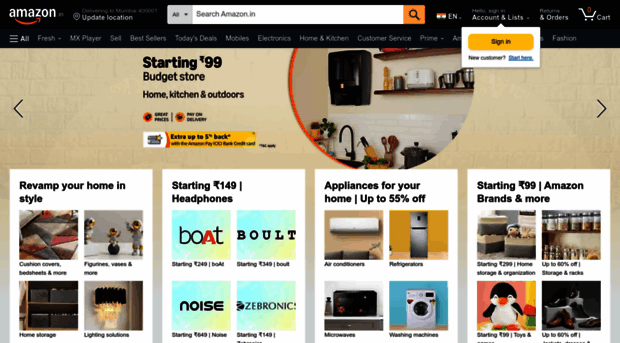The screenshot captures the Amazon homepage. At the top left corner, it prominently displays the Amazon logo. Next to the logo, there's a location marker indicating delivery to "Mumbai 400001," with an option below to "Update Location" in white text. Central to the page is a large search bar for easy navigation.

The middle section features a promotional banner encouraging users to "Shop Latest Smartphones," showcasing three different smartphone models. Below this banner, a series of categorized cards offer various shopping options: "Makeup Products," "New Looks for the New Season," "Do Up Your Home," and "Smart Gadgets by Amazon."